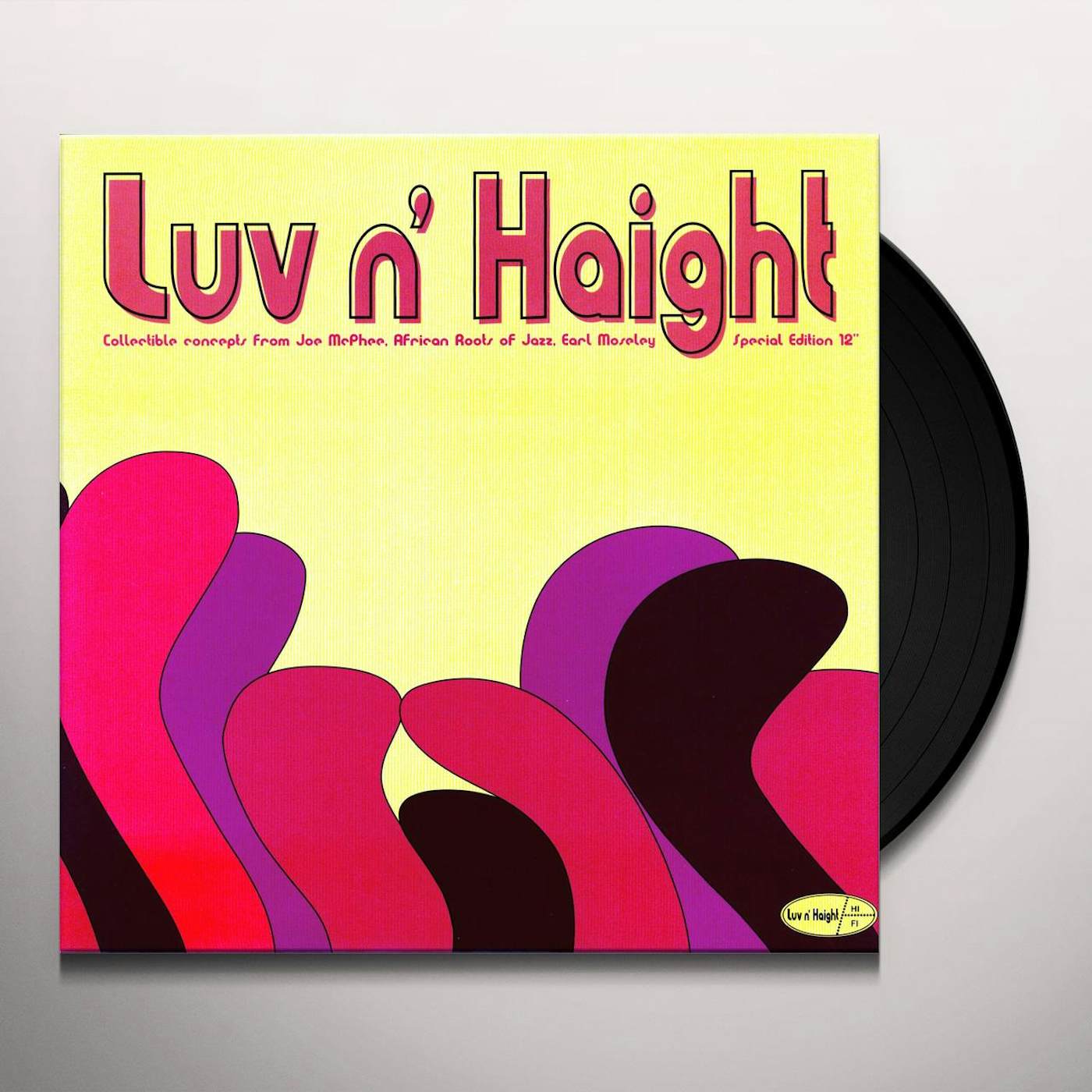The image showcases a collectible vinyl record titled "LUV-N-HEIGHT," with the cover prominently featuring a yellow background and vibrant red text at the top. Below the title, it states: "Collectible concepts from Joe McPhee, African Roots of Jazz, Earl Mosley, Special Edition 12-inch." The vinyl cover is adorned with a dynamic, wave-like design at the bottom, resembling sea kelp, with undulating shapes in shades of black, purple, and red. In the bottom right-hand corner, a small sticker caption reads "LUV-N-HEIGHT HIFI." Peeking from behind the cover, a sliver of the black vinyl record is visible. The entire setup is placed on a beige background with a gradient that becomes grayer towards the bottom.